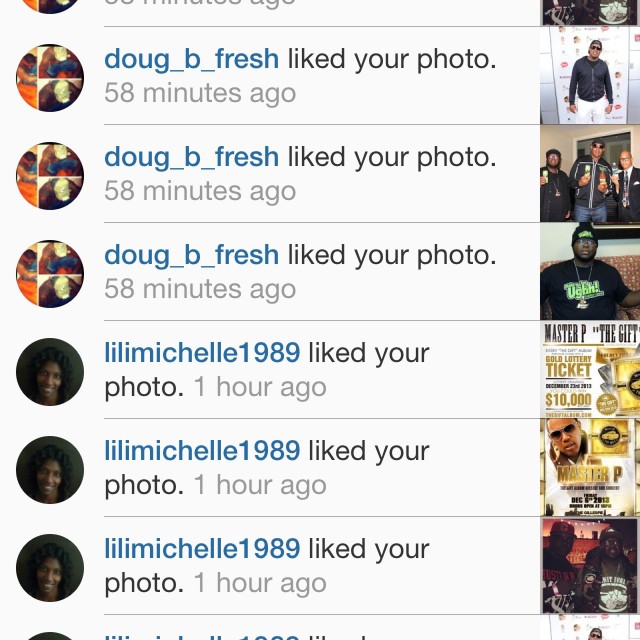The image is a screenshot taken from a social media platform, likely Facebook, showing a series of notifications of people liking the latest photo posted by the user. The likes are primarily from two users: Doug B. Fresh and Lily Michelle 1989. 

On the left-hand side of the screenshot, there are profile pictures representing the people who have performed the actions. In the middle section, it starts with "Doug_B_Fresh likes your photo" repeated several times. The photo associated with these notifications features a black male wearing a backward cap, sunglasses, a black jacket, and white trousers. This central character appears again in a group photo with two other black males, of whom the one in the middle (wearing sunglasses) is the same individual from the initial solo picture. Another notification from Doug B. Fresh is linked to a different image of a black male in a black t-shirt with a red symbol and the word "UGHH" followed by an exclamation mark.

Following Doug B. Fresh’s notifications, the screenshot shows multiple entries indicating that "Lily Michelle 1989 likes your photo", all related to images featuring African American individuals. One is a picture of Master P titled "The Gift", and other notifications repeat with different photos of Master P. There's also a photo of two black males both wearing baseball caps under her likes.

Doug B. Fresh and Lily Michelle 1989 are significant figures in the notifications, both engaging multiple times with a variety of photos, all portraying individuals of African descent.